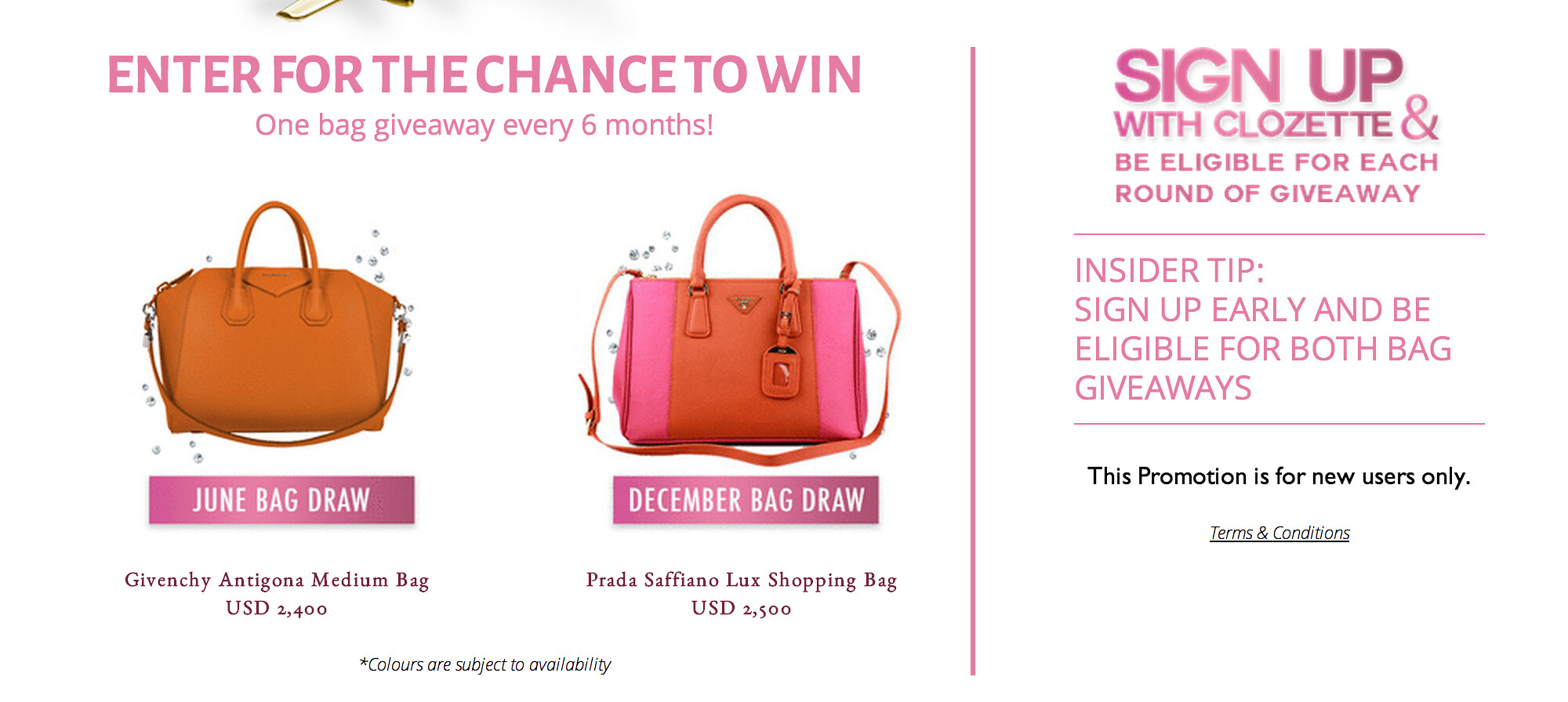The advertisement is a promotion for a sweepstakes from Clozet, displayed on a white background with pinkish purple text. The ad is divided into two sections by a vertical pink line. On the left side, it reads "Enter for the chance to win one bag giveaway every six months" in pink text. Below this, there are two images of handbags. The left image features an orange Givenchy Antigona Medium Bag, valued at USD $2,400, with a pink bar underneath labeled "June Bag Draw." The right image shows a pink and orange Prada Saffiano Luxe Shopping Bag, valued at USD $2,500, with a pink box underneath labeled "December Bag Draw." A small disclaimer below these images, in black text, notes that colors are subject to availability.

On the right side of the pink dividing line, the text states "Sign up with Clozet and be eligible for each round of giveaway. Insider tip: Sign up early and be eligible for both bag giveaways." This section is flanked by lines above and below the text. In black font, it also mentions, "This promotion is for new users only." At the bottom, there is an italicized hyperlink that reads "Terms & Conditions."